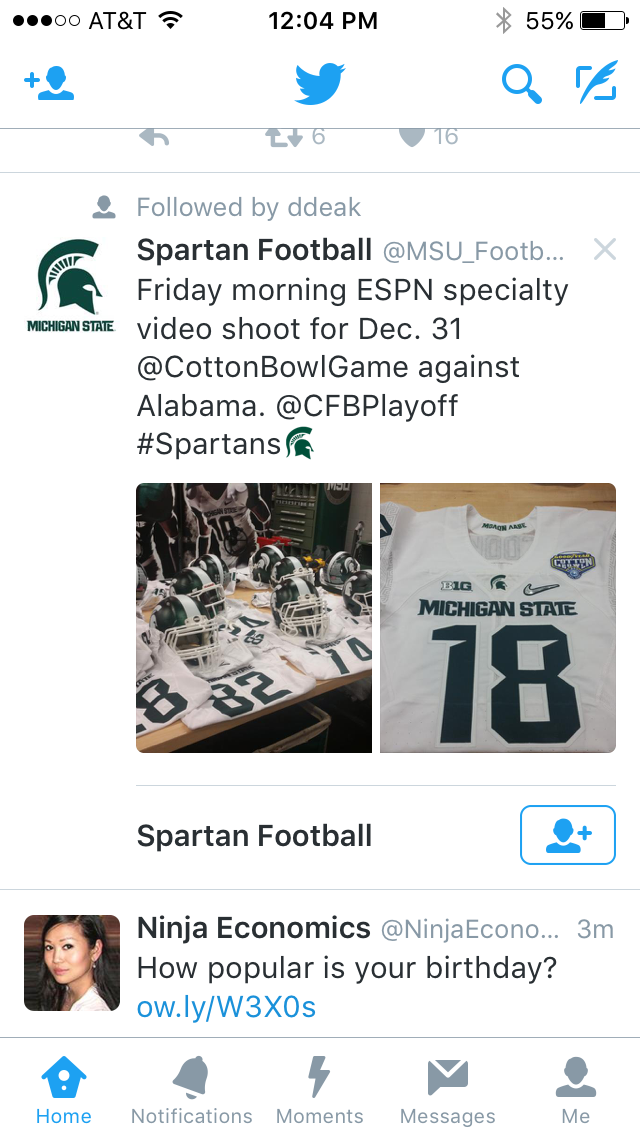This is a detailed screenshot of a Twitter feed on a smartphone displaying the familiar AT&T logo and internet symbol at the top, with the time noted as 12:04 p.m. and a battery life at 55%. Centered on the screen is the iconic blue Twitter bird. Below it, the Michigan State logo, a green Spartan helmet, signifies the account Spartan Football (@MSU_Football). The tweet highlights a Friday morning ESPN specialty video shoot for the December 31 Cotton Bowl game against Alabama, part of the College Football Playoff.

Prominently featured in the middle of the screenshot is an image split into two sections: the left shows a Michigan State Spartan helmet resting on top of a pile of white jerseys, while the right displays a white Michigan State jersey with the number 18 and a Nike logo. Underneath this, in black text, it repeats “Spartan Football.”

Further below, there is a secondary tweet from an account named Ninja Economics (@NinjaEcono) noting "How popular is your birthday?” Finally, at the bottom of the screenshot, the standard Twitter navigation bar is visible, including icons for Home, Notifications, Moments, Messages, and Me.